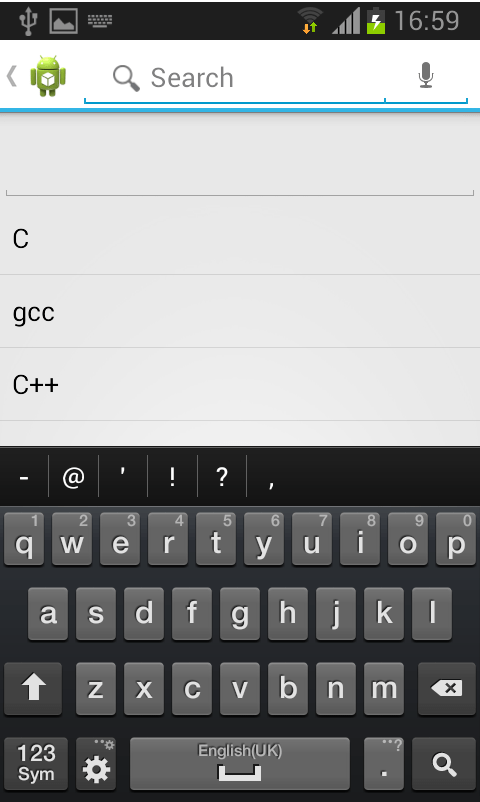The image showcases an Android search interface on a smartphone. In the upper left corner of the screen, there is a USB icon, indicating a connected device. The status bar shows other icons including a photo image, a keyboard, a Wi-Fi signal with four bars, and a battery meter approximately at 50%. The time displayed is 16:59. Below the status bar is a 3D Android logo centered on a white background.

Directly beneath this is a search bar with a magnifying glass icon and the word "search," followed by a microphone icon to the right. This search bar is underscored by a blue line, with an additional solid blue line extending across the screen. Below this, the field transitions to a light gray, containing text entries: "C" on one line, "gcc" on the next, and "C++" on the following line, each separated by thin gray lines.

The lower portion of the screen displays a QWERTY keyboard. The keys are light gray with white letters, set against a medium gray background. Some keys, such as the up arrow, numeric toggle ("1 2 3"), settings gear icon, backspace, and search keys, are slightly darker gray. Above the keyboard, there are dark gray symbols including a dash, at symbol ("@"), quotation mark, exclamation point, question mark, and comma. At the bottom of the keyboard, it reads "English (UK)," indicating the language setting.